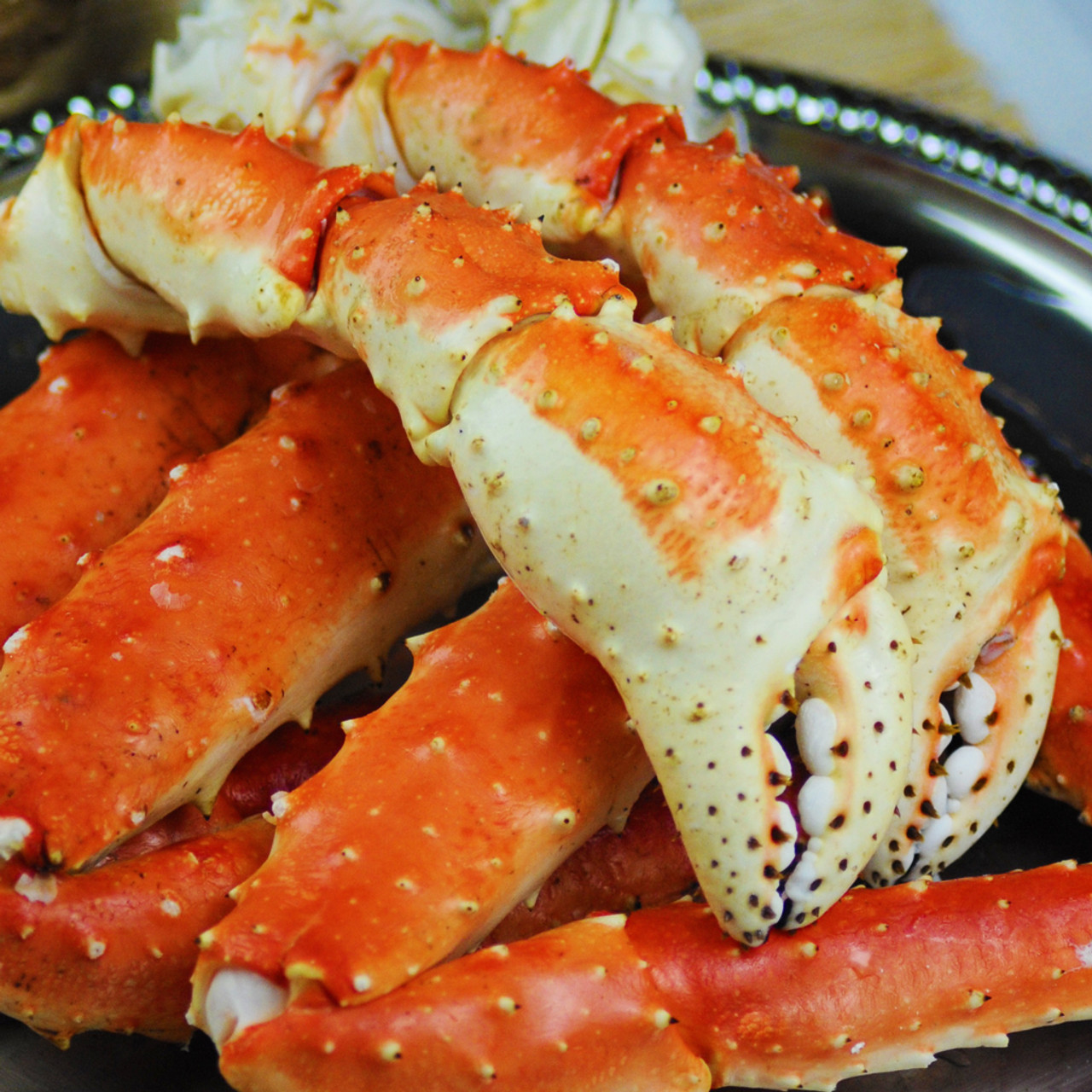This horizontally rectangular, professionally staged indoor photograph is captured from a slight overhead angle using artificial light. The image features a close-up of crab legs displayed on a shiny, dark brown plate with a textured decorative rim. In the upper left and right corners of the image, parts of the brown table are visible, and the upper right corner includes a white placemat, adding context to the indoor dining setup.

The crab legs dominate the composition, showcasing their spiny red exterior with bumps and small brown spots. Some of the legs have been cracked open to reveal the white meat inside. The claws themselves are red on top and white underneath, with small white bubble-like structures that resemble teeth but are not. The crab legs are arranged in what appears to be clusters, suggesting they may have been steamed. The vibrant hues and intricate textures of the crab legs, juxtaposed with the dark plate and furnishings, highlight the detail and appeal of this seafood dish.